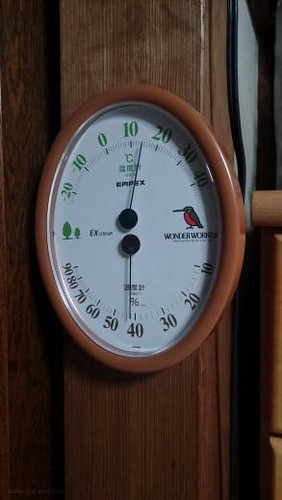The photograph is taken in a dimly lit interior space, capturing a section of a wall adorned with intricately crafted wood molding. The molding, which frames a recessed portion of the wall, is a rich coffee brown color. To the left, a small portion of the wall is visible, continuing the same wood molding design. The right side of the image fades into a dark shadow, suggesting the presence of an open door or a hallway.

Prominently featured on the wall is a large, oval-shaped plastic mount in a similar brown hue. Set within this oval is a white-faced dial, which, at first glance, resembles a clock but is likely a thermometer. The upper half of the dial features red numbers ranging from 20 on the left to 40 on the right, with a small black hand indicating a reading of approximately 12. This section also includes decorative elements—two small trees and a bird on either side of the scale.

Below this, a second similar setup is present, with the scale ranging from 10 to 90. The indicator on this lower part shows a reading of approximately 43. The overall design and elements suggest that this instrument may be a combined thermometer and hygrometer, used for measuring temperature and humidity.